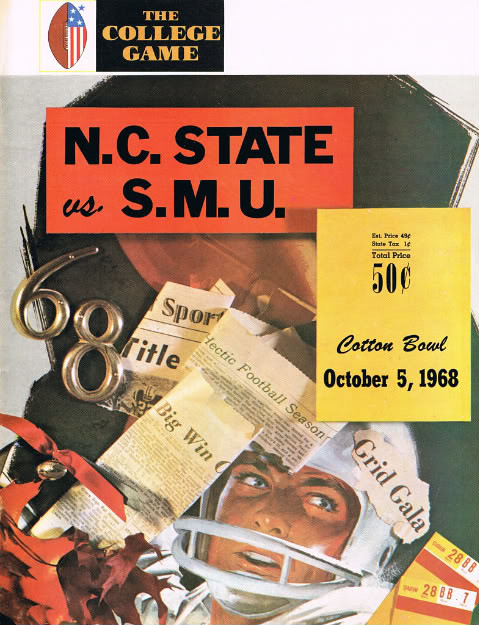The image is a detailed collage poster for a historical college football game between NC State and SMU, dated October 5th, 1968. The top of the poster features an image of a half brown, half American flag-colored football, and a black rectangle with yellow or orange letters that read "The College Game." The background of the poster is a vibrant collage that includes an illustration of a man wearing a white football helmet, various newspaper clippings with phrases like "Grid Galar Big Win Sport" and "Hectic Football Season," and red leaves. Prominently displayed is a gold number "68." Additionally, there are two tickets in yellow, red, and white colors situated on the bottom right. A red rectangle with black text reads "NC State vs. SMU," alongside a yellow rectangle proclaiming, "Total Price, 50 cents, Cotton Bowl, October 5th, 1968."